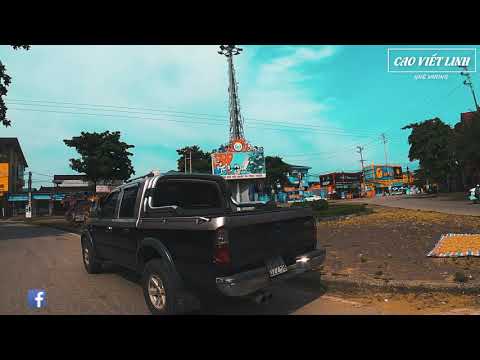The image depicts a black pickup truck positioned nearly at the center of a small, dirt-covered road devoid of lane markings. To the right of the truck lies a concrete curb adjacent to a dark brown dirt patch. The background features a prominent cell phone antenna with lights at the top and an attached billboard displaying orange, light blue, and dark blue hues. Brightly colored multi-storied buildings serve as a vivid backdrop; notably, a light blue building occupies the left center, with a red and black building nearby and an orange and blue building further to the right. Overhead, the light blue sky is dotted with white clouds and intersected by power lines. Additionally, trees are visible amid the buildings and other structures. Notable elements also include the Facebook logo in the bottom left corner and some text, "KO Viet Lin," seen in the upper right, lending an impression of a lively, possibly Mexican, outdoor setting captured in the middle of the day.